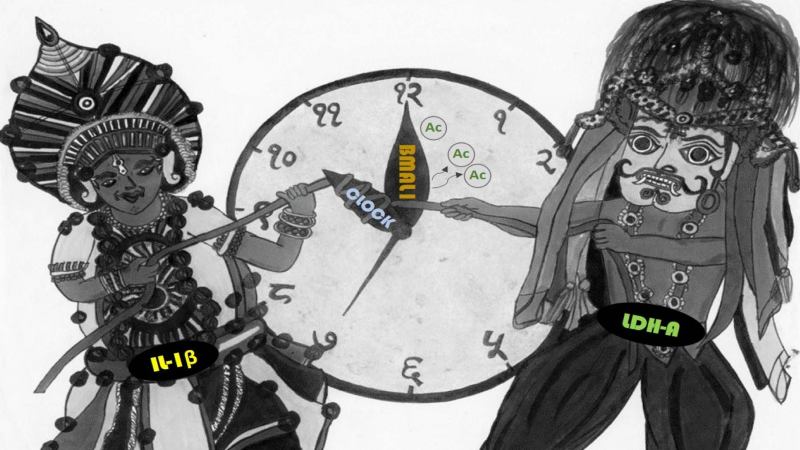This hand-drawn image, primarily in black and white with some colored accents, features two figures on either side of an unusual clock. On the left is a woman wearing a large, multi-layered turban resembling a flame at the top, and she's dressed in a decorative outfit. She holds a guitar-like instrument and has a black oval at her waist with yellow letters reading "I-I-B." On the right stands a man with a curly mustache and a large turban. He wears a black shirt and pants, and has an oval at his waist with green letters spelling "L-D-H-A." Both figures are tugging on a rope wrapped around the clock's hands. This clock is peculiar, with numbers arranged whimsically: "92" at the top, followed by "9", "2", and then obscured segments showing "Y", a backward "3", "6", "5", another backward "9", "90", "99," and back to "92". The minute hand is labeled "B-M-A-L-I" in orange, and the hour hand has "clock" written in light blue letters. The seconds hand is unlabeled. The image is a complex melding of artistic whimsy and intricate detail, highlighted by the dynamic tension between the two figures and their mysterious clock.